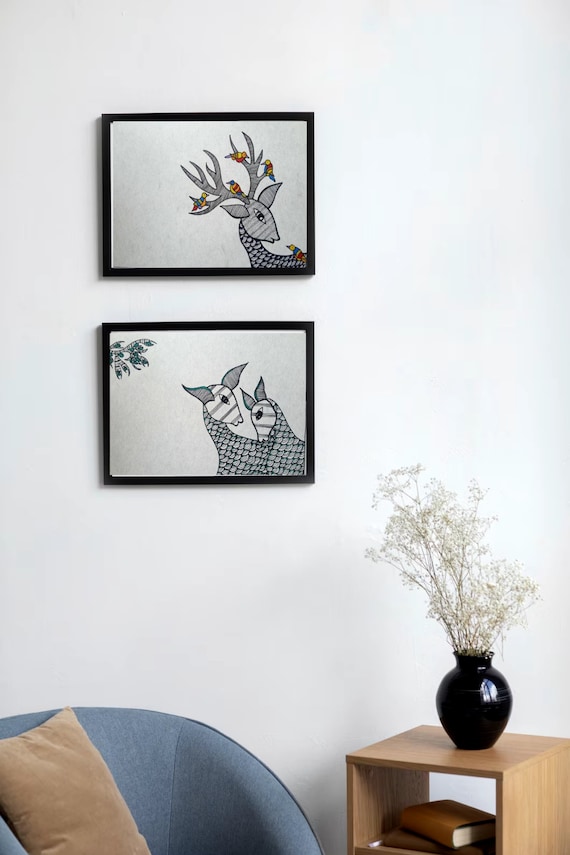The photograph captures a serene living room setting dominated by a white wall adorned with two horizontal, rectangular paintings framed in thin black frames. The top painting features a stylized drawing of a dark gray deer with four colorful birds perched on its antlers and one on its body, imparting a whimsical touch. Below it, the second painting depicts two deer heads in the lower right corner, incorporating white heads and green leaves in the top left corner, adding a subtle pop of color. In the lower left of the frame, part of a blue couch is visible, accented with a beige or tan pillow that adds a comforting contrast. Adjacent to the couch, a small, wooden table with an open shelf holds two books—one with a brown cover and another with an orangey-brown cover. On top, a shiny black vase houses delicate white flowers, likely baby's breath, contributing to the room's understated and minimalist decor. Light, possibly sunlight streaming through a window, enhances the calm and inviting atmosphere of the room.